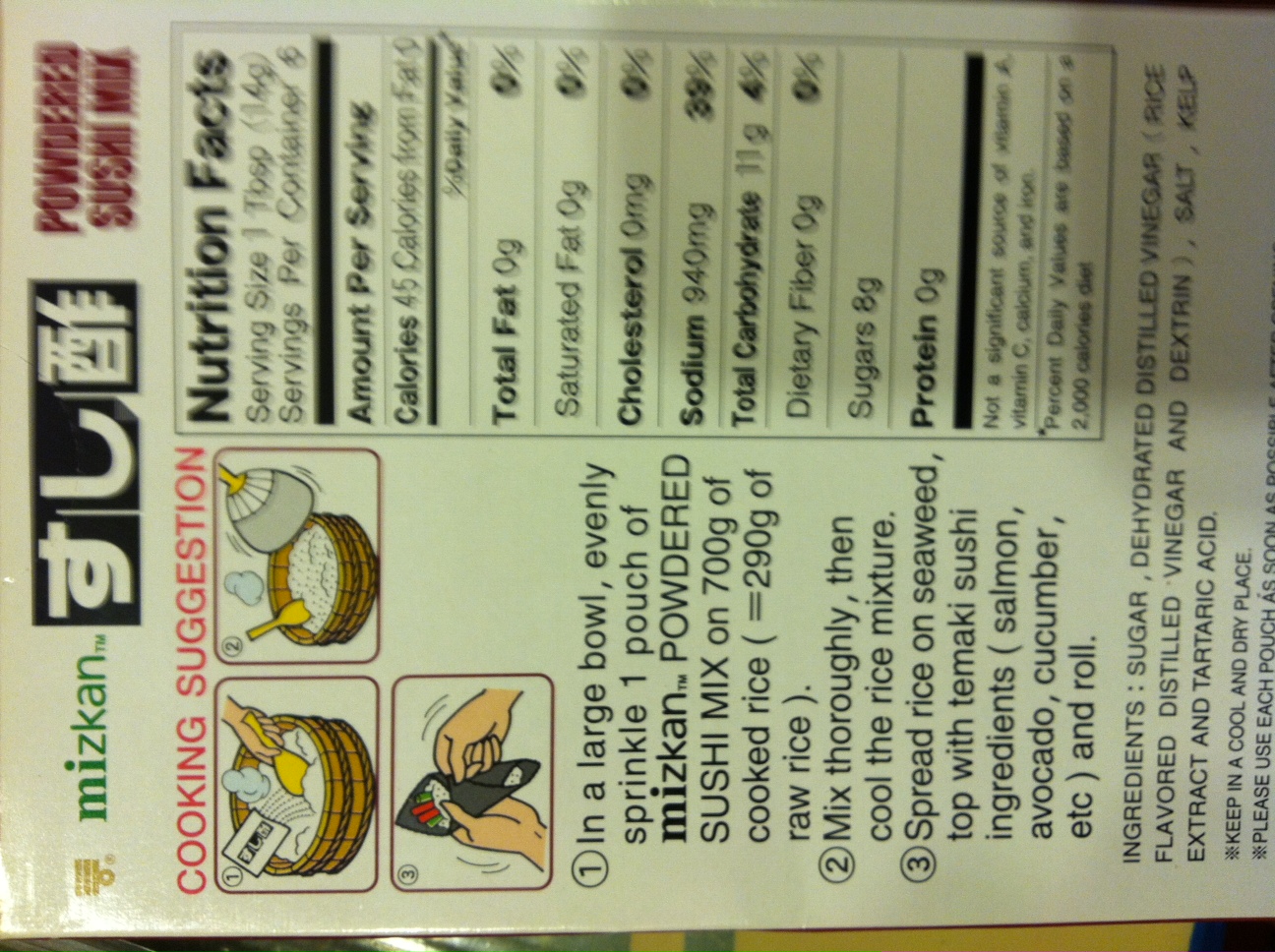This image captures the back of a powdered sushi mix packet, marked by the prominent red text “Powdered Sushi Mix” at the top right. The green label, “Ms. Can,” is displayed at the top left, alongside some Japanese characters in black and white at the top center. The right side of the photo, slightly blurred, contains a white and black nutrition facts panel. The central area features three color-illustrated panels, depicting step-by-step preparation instructions with accompanying text in capitalized red letters under the heading "Cooking Suggestions." Step one instructs to evenly sprinkle one pouch of Ms. Can's powdered sushi mix over 700 grams of cooked rice in a large bowl, mix thoroughly, and then cool the mixture. Step two indicates to spread the rice on seaweed, and step three describes topping with ingredients like salmon, avocado, cucumber, and then rolling the sushi. At the bottom, a list of ingredients is noted in black writing. The image, taken by a cell phone or personal camera, also shows a slight camera shadow, hinting at an informal capture.